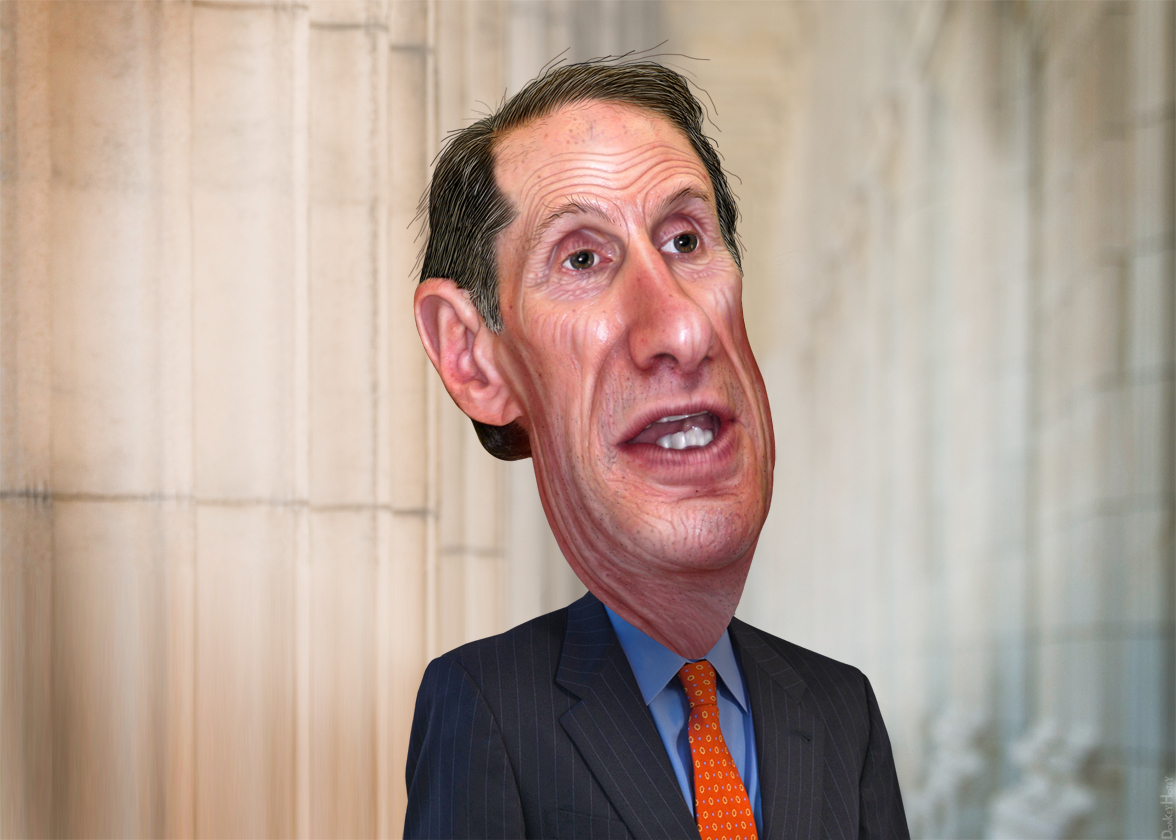This horizontally-aligned rectangular image depicts a man in a business suit with a somewhat distorted, puppet-like appearance. He has an elongated face with raised eyebrows and numerous wrinkles etched along his cheekbones and forehead. The man’s brown eyes look wide open, and his mouth is agape, revealing a set of crooked but white bottom teeth. He is dressed in a subtly striped black suit jacket with gray stripes, paired with a blue collared shirt and a striking orange-and-white patterned tie.

The background of the image is somewhat blurred, particularly on the right side, creating a blend of brown and white colors. However, the left side is more discernible, showcasing what appears to be a wall crafted from vertical, rectangular stone sections in a light brown hue. This provides a stark contrast to the indistinct, blurred portion on the right, adding an intriguing element of depth and texture to the overall composition.